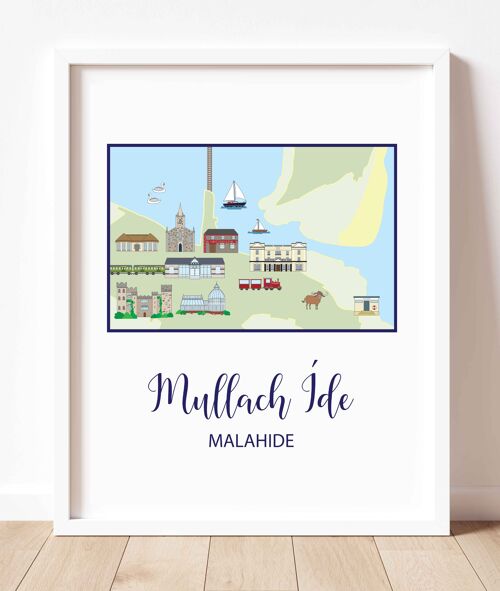The photograph features a white-framed picture leaning against a white wall on a whitewashed wooden floor composed of planks. The picture inside the frame is a detailed, hand-painted map of the town of Malahide, and it is bordered in blue. The map exhibits a charming folk art style with various simplistic yet intricately detailed buildings, including a stone church, a school, a possible hospital, a small castle on the outskirts, and a trolley train with an engine and two cars. Water elements are prominent, with a couple of sailboats to the right side, a large and a smaller one navigating near the railroad line that extends out to sea, and ducks swimming nearby. Notably, a cow is also depicted within the town. Below the drawing, "Malachide" is written in elegant cursive blue lettering, with "Malahide" printed in regular blue font underneath, suggesting the name in different script forms or languages.